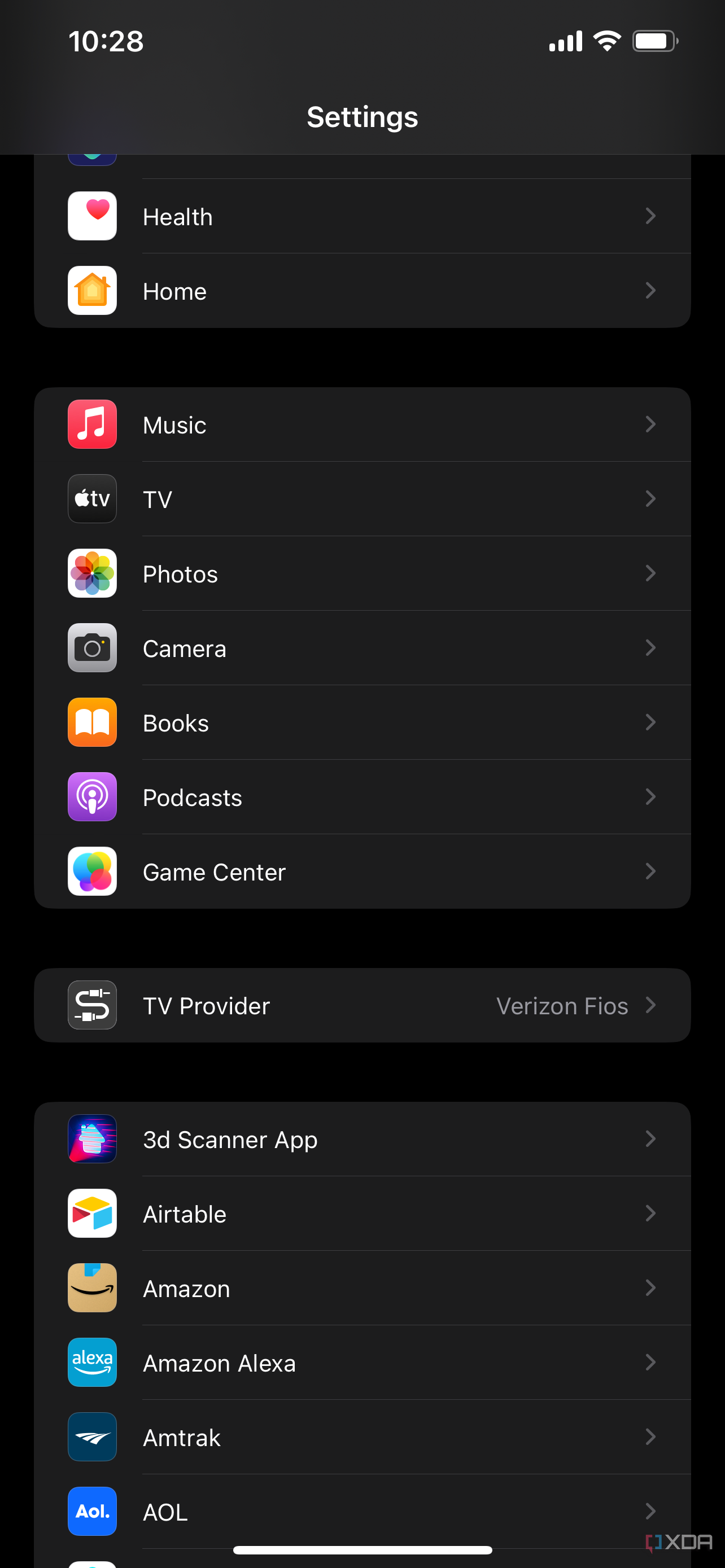A detailed caption for the image could be:

---

An iPhone displayed in dark mode, showcasing the Settings menu with a variety of apps listed alphabetically. The visible portion of the list includes system apps and third-party applications such as Health, Home, Music, TV, Photos, Camera, Books, Podcasts, Game Center, TV Provider, 3D Scanner App, Airtable, Amazon, Amazon Alexa, Amtrak, and AOL. Each application is accompanied by a relevant icon: Music has a double musical note, Camera features a camera icon, Books shows an open book, and Podcasts displays a broadcasting antenna. The TV Provider section indicates Verizon Fios as the selected provider. At the bottom-right corner, there is a watermark labeled "XDA," typically associated with Android devices, implying the possibility of a custom ROM or operating system that mimics the iPhone interface. The notification bar at the top reveals a battery level at 90%.